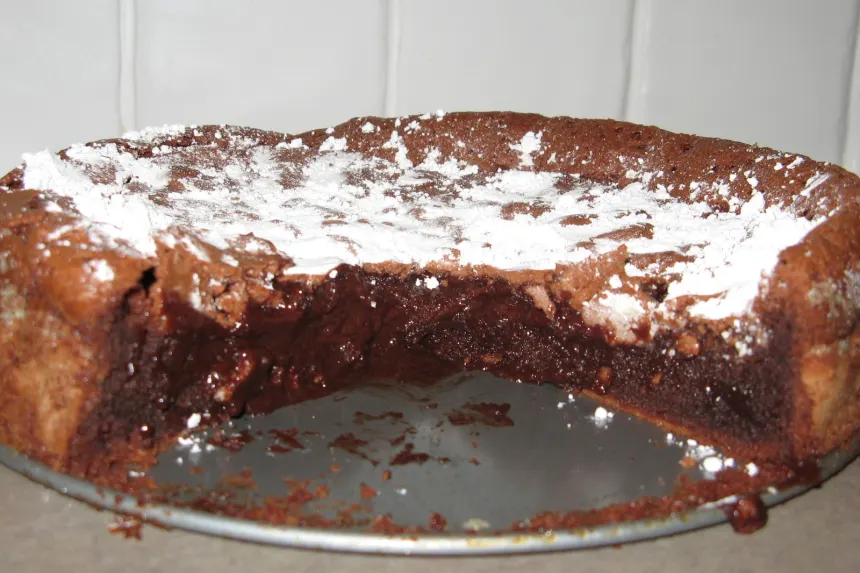This close-up photograph captures a large, somewhat messy chocolate dessert on a tin pan. The dessert resembles a molten lava cake with a gooey, almost liquid-like chocolate center and a cakey outer layer. The rich, moist chocolate inside oozes out, contrasting with the slightly overdone and less rich edges. A substantial portion of the cake has already been eaten, exposing its uneven, soft interior. There are slices missing, revealing areas flooded with chocolate and scattered with what appear to be bits of nuts. The top of the cake is heavily dusted with powdered sugar, more than for mere decoration, giving it a dense, snowy appearance. The tray underneath is littered with crumbs, and the surface upon which the tray rests is gray. The background features a white paneled wall with five panels, adding to the overall homely yet untidy feel of the scene. The dessert, despite its luscious interior, looks somewhat unappealing due to its raw-like center and overdone edges.